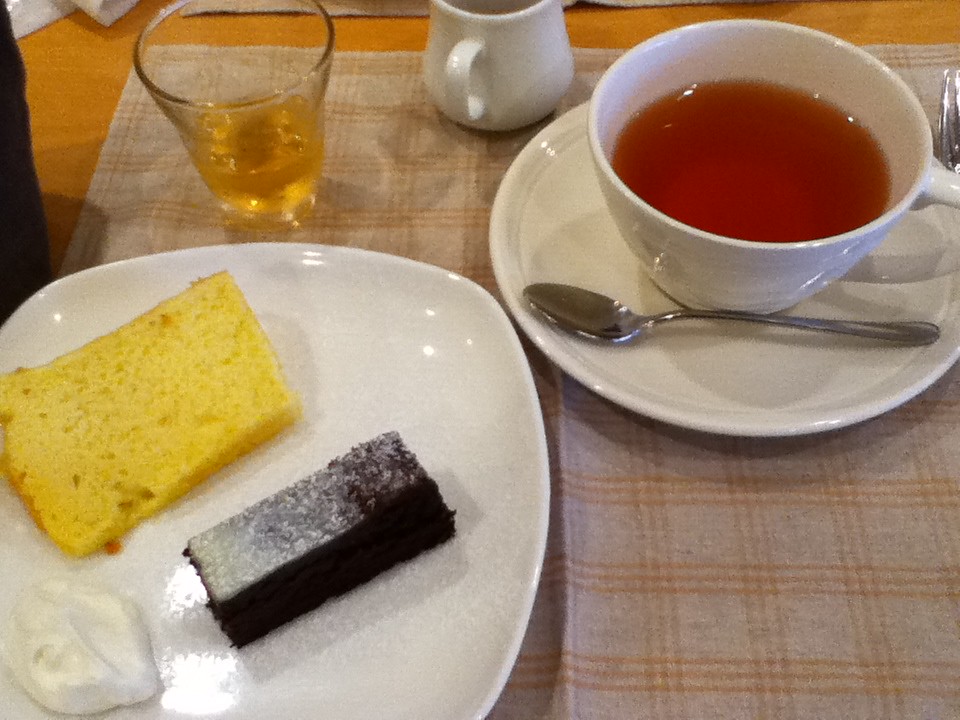The image depicts a meal at a diner, showcased on a light-colored wooden table adorned with a tan and light brown striped tablecloth. Centered in the photo is a small, white, square plate featuring a slice of yellow sponge cake, a thin piece of chocolate brownie, and a dollop of whipped cream. To the right of the plate is a small, white teacup filled with tea, resting on a saucer with a silver spoon beside it. Positioned slightly to the left is a small glass, containing a third of yellow-orange liquid, presumably orange juice. Adjacent to the glass is a white creamer container. The table setting exudes a cozy, rustic diner atmosphere.